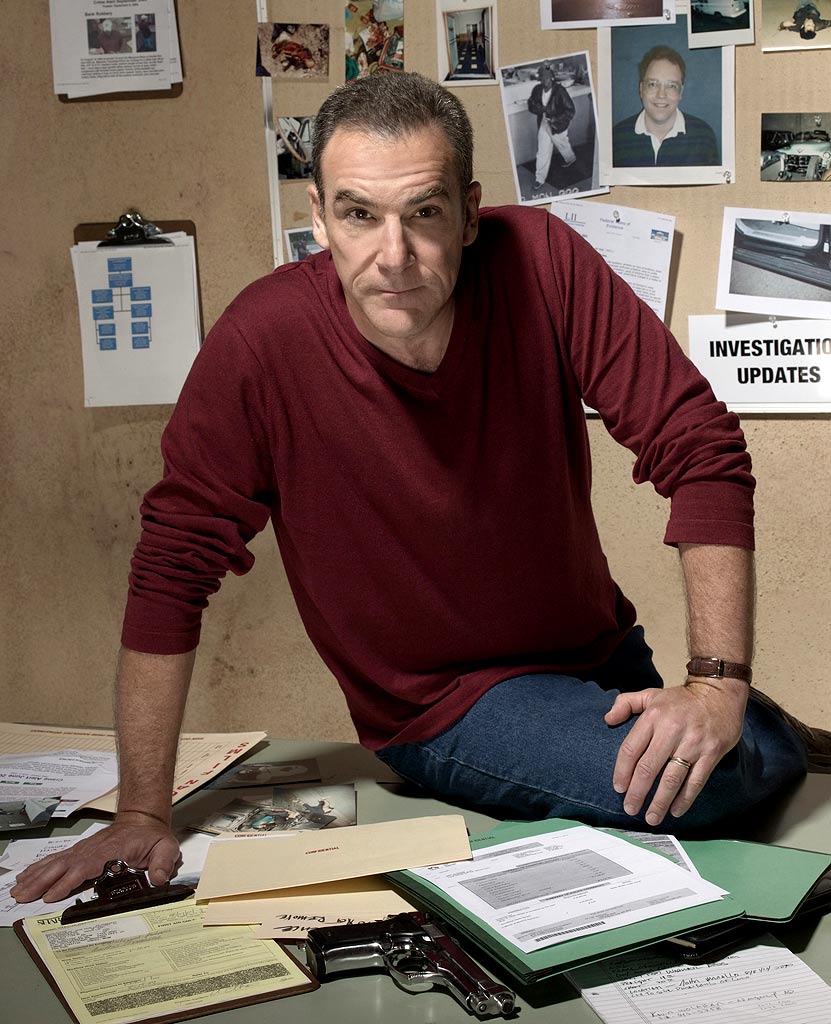In the photograph, a caucasian middle-aged man with short, receding dark hair sits on the edge of a gray-green desk, gazing intently into the camera. Dressed in a long-sleeved burgundy V-neck shirt and blue denim jeans, he exudes a serious demeanor, with lines of concentration on his forehead. His left hand rests on the desk while his right hand is placed on his knee, revealing a brown leather wristwatch on his left wrist. The desk is cluttered with various papers, manila folders, green files, and a clipboard, among which a silver metallic handgun is conspicuously placed, pointing off to the side. Behind the man, the dirty wall is adorned with numerous photographs, charts, and papers pinned to clipboards, alongside a bulletin board overflowing with images. A white sign at the bottom of the board reads "Investigation Updates," suggesting a detective or law enforcement context.